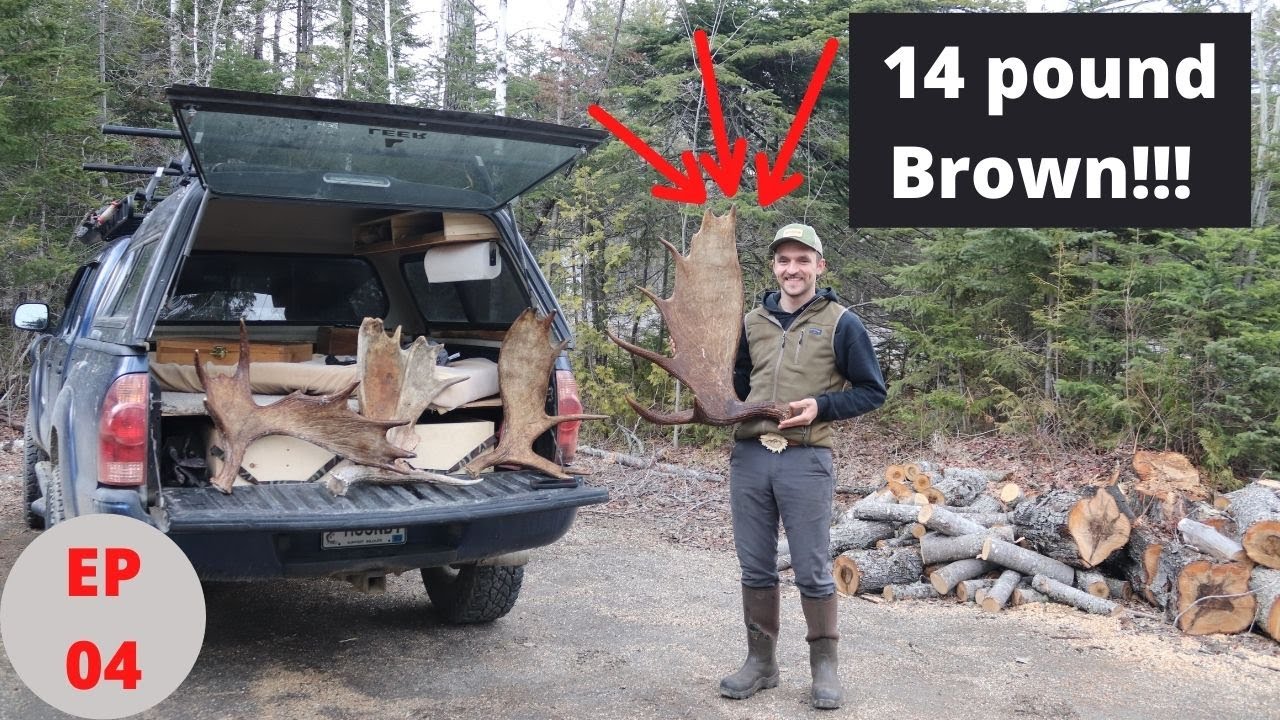In this daytime photograph, a man stands smiling at the camera in a forested area, dressed in a green cap, gray trousers with knee-length gumboots, a hoodie, a long-sleeve dark blue shirt, and a half-green jacket. He is holding a large moose antler. Behind him, a gray van with its tailgate down and hatch up reveals multiple large moose antlers in the open bed. 

On the right side of the man, chopped wood piles along the road hint at recent logging activity. The background is filled with trees, some of which appear to have been cut down, adding to the rugged, natural setting. At the bottom left of the picture, a gray circle with red letters reads "EP04" or "episode 4." In the top right corner, a black rectangle with large white text reads "14 pounds brown." Above the antlers in the van's bed, three red arrows are pointing towards them, emphasizing the focal point of the scene. 

The details combined highlight an outdoor, forest environment with a van and a man prominently showcasing moose antlers, hinting at a hunting or wildlife theme.